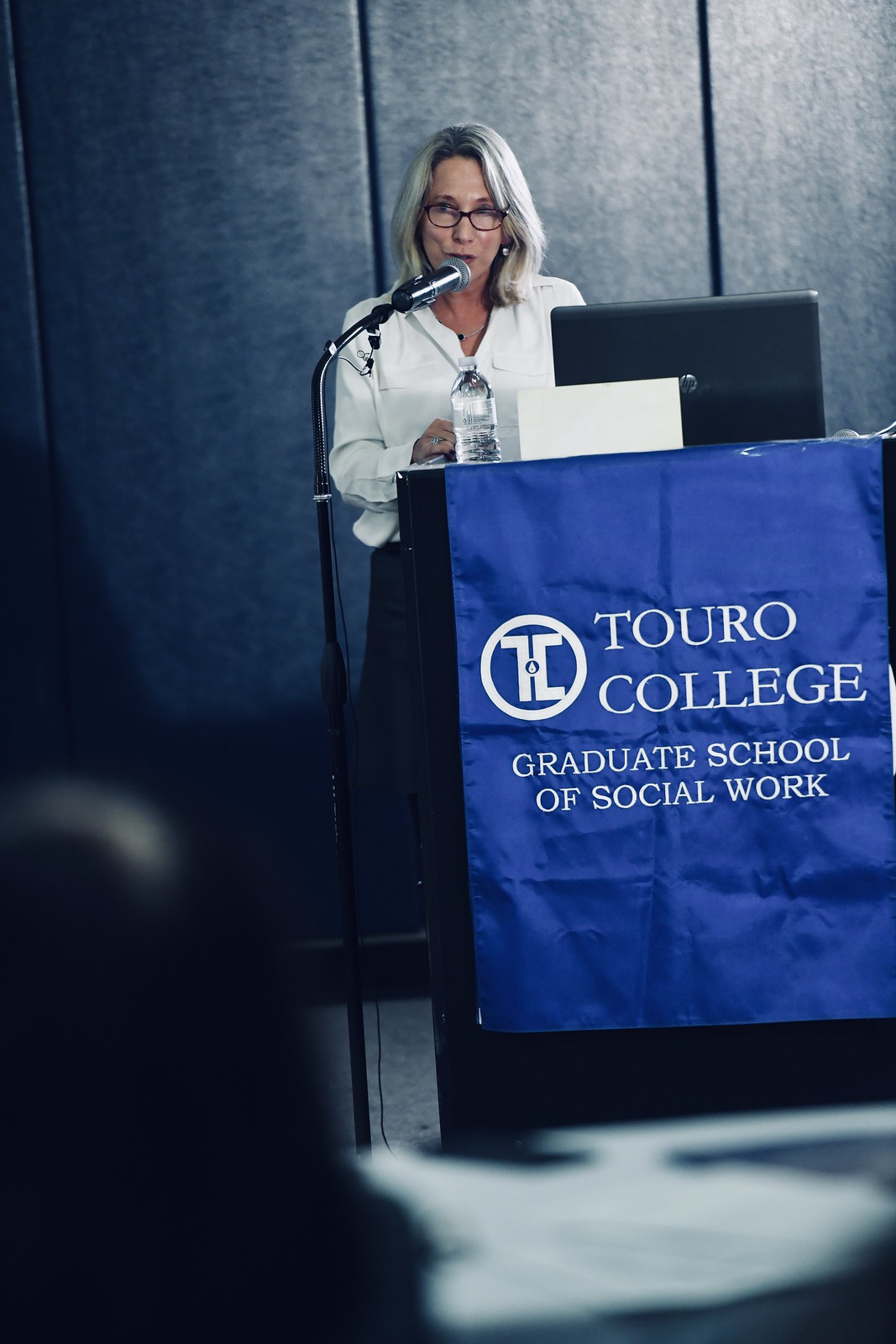In the image, a woman stands behind a rectangular, boxy podium, speaking into a microphone. The woman is visible from her waist upwards, wearing a white button-up blouse adorned with a chest pocket and shoulder loops. Her blouse has long sleeves with zippers currently zipped up. A black, slightly curved microphone holder with a black microphone, which features a round silver ball, extends towards the woman's face. She has shoulder-length gray hair and is wearing brown-rimmed glasses. The podium prominently displays a blue flag with white text that reads, "Touro College Graduate School of Social Work." Additionally, a black HP laptop and a water bottle are placed on top of the podium. Behind the woman, the wall appears to be either black or dark blue with light reflecting off the top right corner.